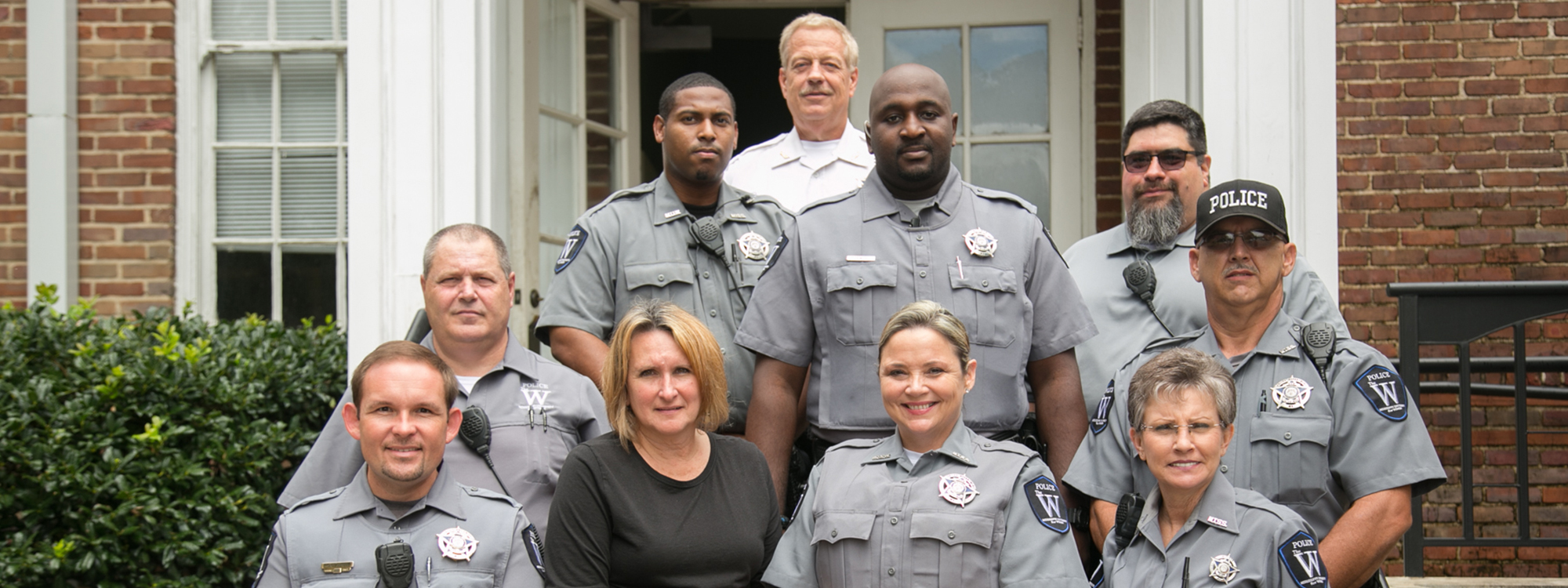This horizontally-aligned photo features a group of police officers posing for a group picture in front of a brown and white brick building. The building's façade includes two doors; the left one is open, and the right one is closed. To the left of the group, there's a bush that appears to be hollies, while a metal railing is situated to the right. Most of the officers are clad in gray, short-sleeved, collared button-down shirts with police badges on their left chests. One officer, positioned on the far right, wears a black cap emblazoned with the word "POLICE" in large letters. In the lower left side of the image, a woman with short blonde hair is not in uniform; she's wearing a black t-shirt. The group comprises three women and several men, with all but two men and one woman in uniform. The officers' expressions range from smiling to serious. The building behind them is characterized by its white trim and window-pane doors.